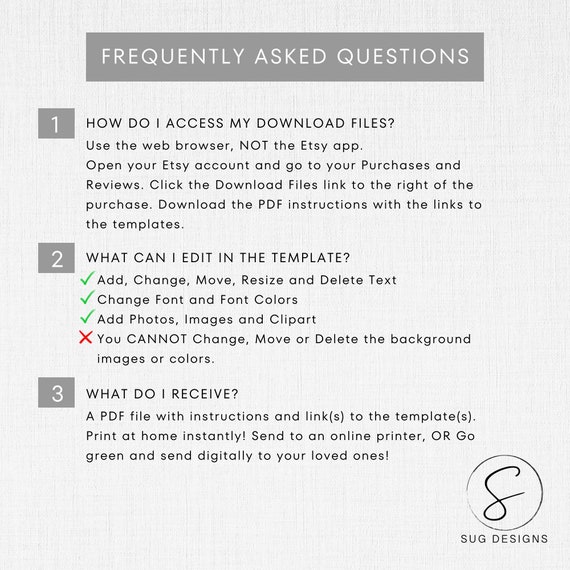This image shows a web page designed as a Frequently Asked Questions (FAQ) section. At the top of the page, within a gray header panel with bold, white text, it prominently displays the heading "Frequently Asked Questions." Below the header, three sections are distinctly outlined in gray boxes, each labeled with white numerals: 1, 2, and 3.

**Section 1**, titled "How do I access my download files?", includes a detailed guide instructing users to use a web browser instead of the Etsy app. It instructs users to log into their Etsy account, navigate to their purchases and reviews, and follow additional steps to access their files.

**Section 2**, titled "What can I edit in the template?", features a list with three items marked by green check marks indicating editable elements and one item marked with a red X indicating a non-editable element.

**Section 3**, titled "What do I receive?", contains a paragraph explaining the contents of a received file, particularly highlighting the reception of a PDF file.

At the bottom right corner of the page, there is a logo inside a circle, which features a stylized figure resembling the number 8, accompanied by the text "sug designs." The overall design uses gray tones for blocks and text, creating a clean and organized layout aimed to help users navigate their queries effectively.